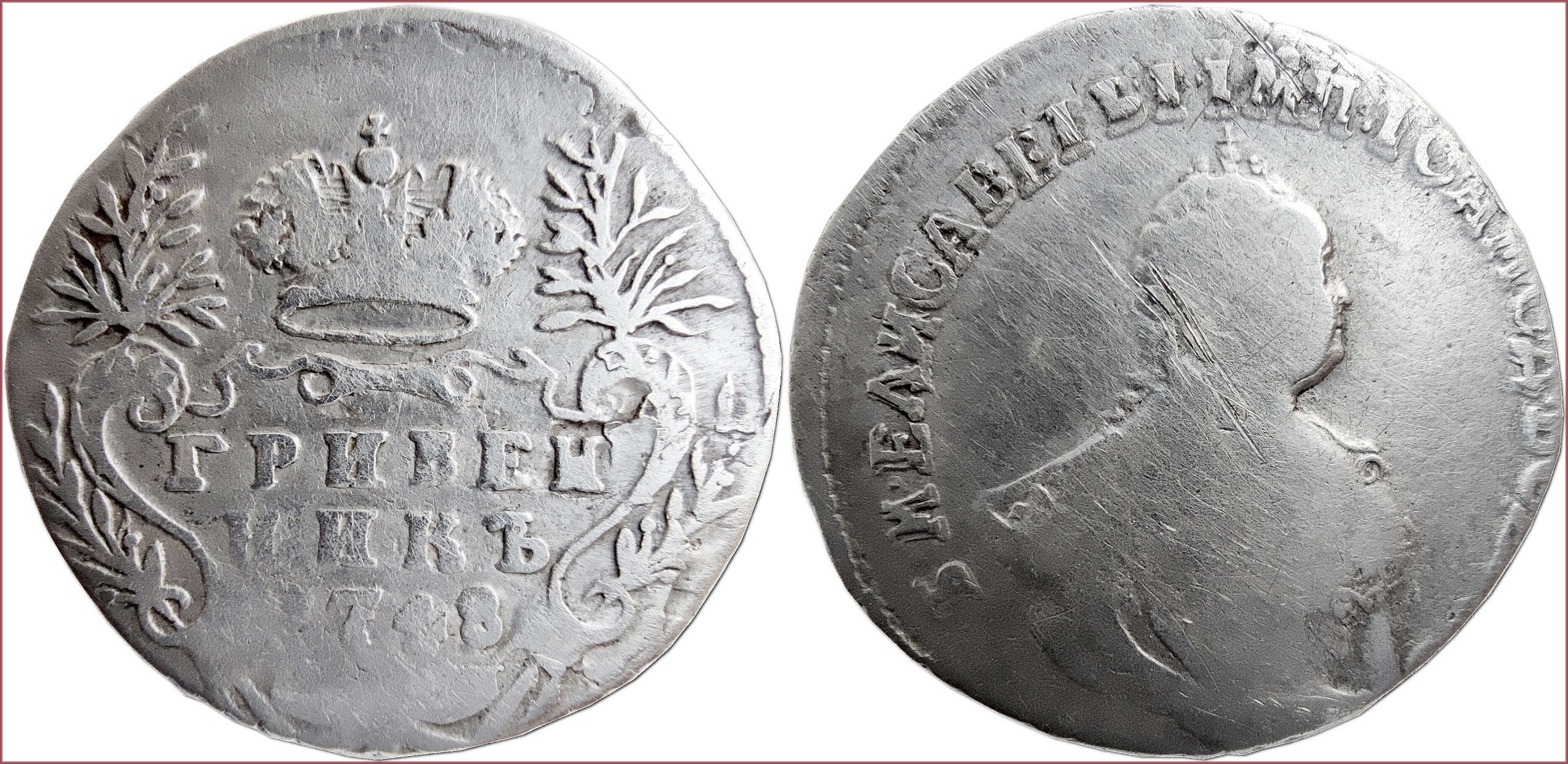The photograph in landscape orientation provides a detailed, black and white close-up of an antique coin, showcasing both its obverse and reverse sides. The left side of the image captures the reverse of the coin, which features a well-defined crown symbol with a small cross at its top center. Beneath the crown, several lines of text can be seen, though they are illegible due to the foreign language and wear. Surrounding the text are curved scrolls or plant motifs. At the bottom of this side, the year 1748 is inscribed, indicating the coin's significant age. The right side of the image shows the obverse of the coin, which is slightly off-center and worn. It displays the distorted profile of a person's face, possibly a queen or notable figure, with circular text around the upper perimeter, also rendered unreadable by wear and the foreign script. The coin itself exhibits slight imperfections and notched nicks, evidencing its antiquity. Both sides of the coin are set against a white background framed by a dark brown line. The overall clarity of the photograph is high, with ample lighting accentuating the coin's intricate details, which are diminished only by time and heavy use. The coin, seemingly from the Russian Empire, offers a fascinating glimpse into history through its representational realism.